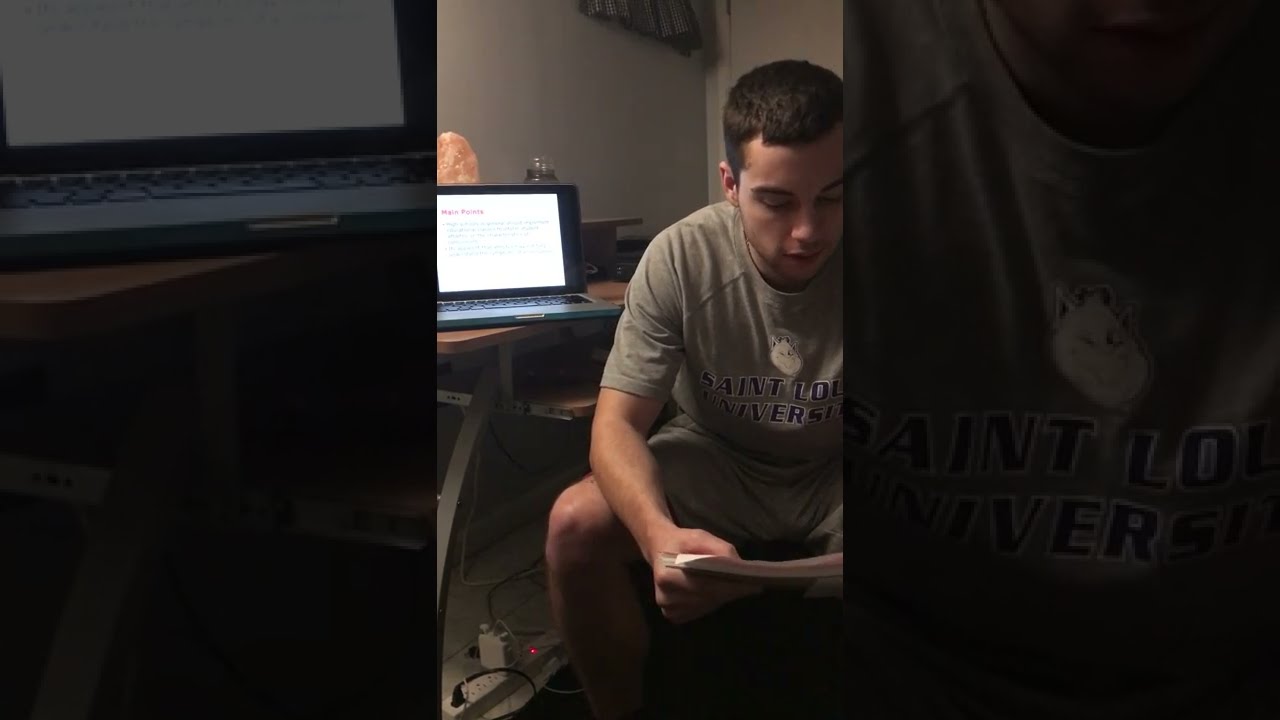The image is a wide rectangular shot featuring a central tall rectangular photograph of a young man reading. This photograph occupies the middle of the image with black bars on both sides. The young man, seated in a chair visible from mid-calves upward, is positioned in the right half of the photograph. He is wearing a light gray t-shirt with "St. Louis University" printed in blue text outlined in white, along with a logo above the text, paired with gray shorts. With a faint mustache and beard, and brown hair, his head is bowed, eyes focused on a notebook or book in his hands, with his mouth slightly open as if reading aloud. His right leg angles towards the left side, supporting his right elbow. 

To his left stands a light brown wooden desk with grey metal supports, on which rests an open laptop displaying a white PowerPoint slide with black text. Behind the laptop is an orange crystal lamp and a glass jar. The desk placement and personal items suggest the setting might be a bedroom or a college dorm.